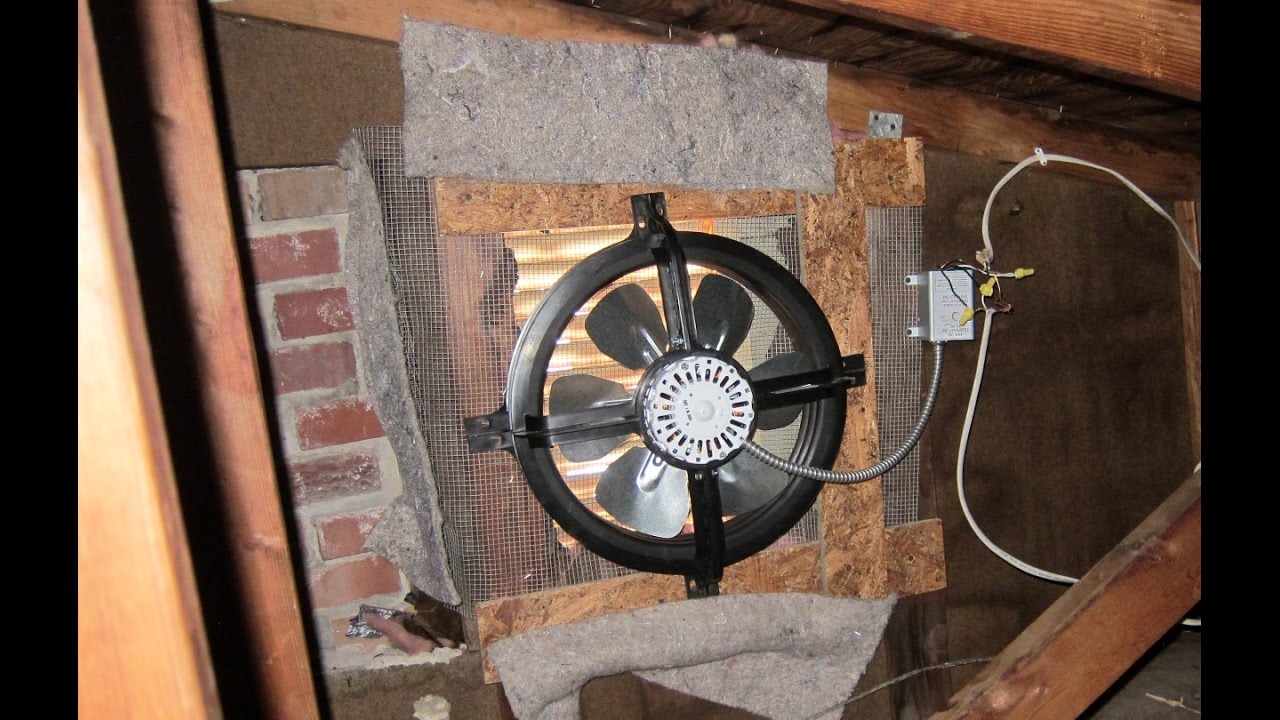The image depicts an unfinished attic with a ventilation fan installed in a somewhat haphazard manner. The fan, which is black with six blades, is mounted to a window to expel hot air, as evident from its orientation. Black brackets support the fan, and the motor, visible from the backside, is a grayish color. It is electrically connected to a junction box via an array of wires. The attic area features exposed red brick masonry on one side and brown particle board on the other, interspersed with some wooden beams. Insulation strips cover some cracks, suggesting attempts to manage the space's thermal efficiency. Moisture stains are visible on the wood, hinting at possible water ingress. The setup includes four wooden blocks of varying lengths helping to hold the fan in place. Overall, the setting is a mix of rustic and functional elements, with some taped-on screen material adding to its makeshift appearance.